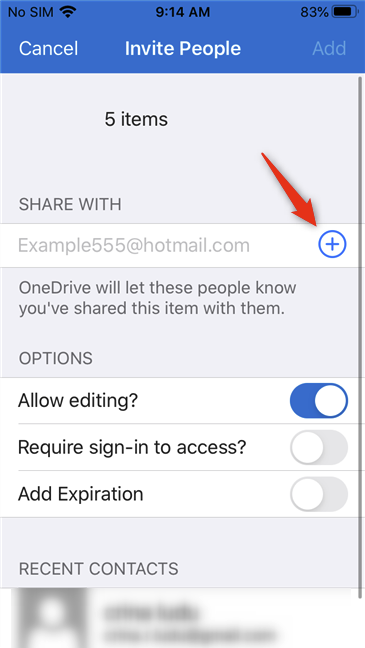This image depicts a mobile app interface, specifically a section of the Facebook app. The top portion of the screen shows standard status icons, indicating there is no SIM card in the phone. It shows a strong Wi-Fi signal, the time at 9:14 a.m. centered at the top, and a battery at 83%. Directly below these status icons, on the app's navigation bar, sits a "Cancel" button on the left, an "Invite People" label prominently in the center, and a grayed-out "Add" button on the far right.

The main interface below features a gray background divided into various interactive elements. The upper section is divided into five items, immediately followed by a "Share with" box that includes a plus symbol, allowing users to add people or email addresses for sharing purposes. Accompanying this box is a note stating, "OneDrive will let these people know when you've shared this item with them."

Further down are three toggle options, each labeled with its respective functions: "Allow editing," "Require sign in to access," and "Add expiration." Each option is accompanied by sliders to enable or disable the features. The bottom section of the screen appears to list recent contacts, although this part is blurred out.